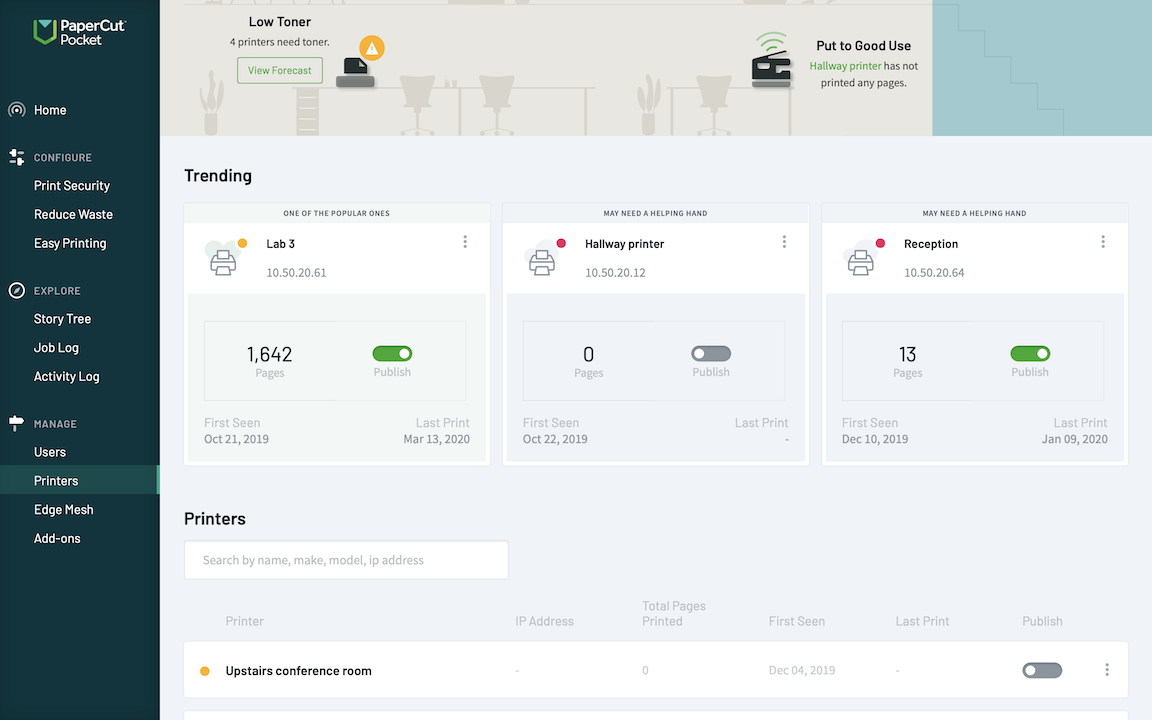A detailed summary of the image shows a notifications panel for a printer:

At the top of the panel, there is a message in bold stating "Low Toner for Printer - Need Toner." Next to this message, there is an orange circle with a white triangle and an exclamation mark inside it, indicating an alert or warning. To the right of this alert, another message reads, "Put to good use - Hallway printer has not printed any pages."

Below, on a light blue background, there is a section labeled "Trending." It lists one of the popular printers as "Lab Printer (IP: 10.50.20.61)," followed by a dark gray or light gray box indicating that this printer has printed 1,642 pages. Next to this box is a green toggle switch turned to the right with the label "Publish." Directly underneath it, additional details show: 
- "First Seen: October 21, 2019"
- "Last Print: March 13, 2020"

On the right side of the panel, there is a section for another printer labeled "Hallway Printer (IP: 10.50.20.12)," which shows it has printed zero pages. This section features a toggle switch above the word "Publish," which is turned to the left and grayed out, indicating that publishing is disabled for this printer.